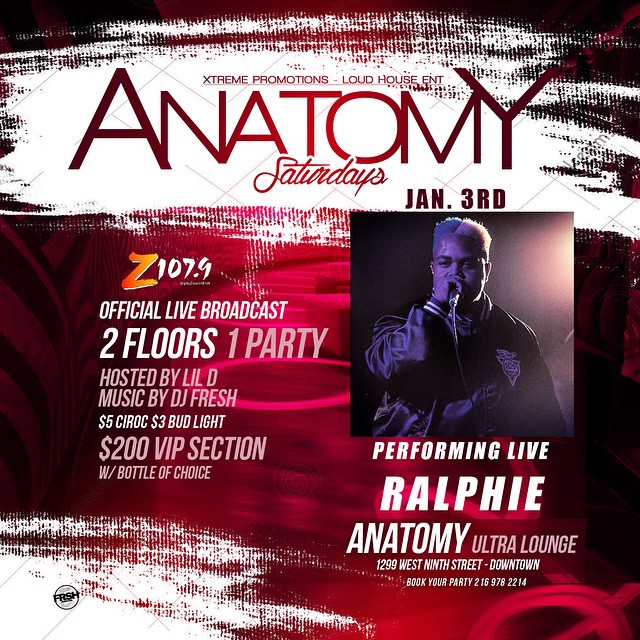The image showcases a flyer for an event called "Anatomy Saturdays," dominated by various shades of red in the background with decorative pink swirls and a white streak forming a banner at the top. The flyer highlights the following details in an organized manner:

At the top, in red text, it reads "Extreme Promotions, Loud House ENT," followed by "Anatomy" in a large crimson uppercase font, occupying around 10-15% of the image height. Below this, in a smaller cursive style, it mentions "Saturdays, January 3rd" in red. The background transitions from dark red to light red, complemented by white and pink decorative swirls. 

On the left side, the flyer features the logo and details of the radio station Z107.9, including "Official Live Broadcast, Two floors, one party" hosted by Lil D, with music by DJ Fresh. It lists the event prices as "$5 Ciroc, $3 Bud Light, $200 VIP section with a bottle of choice."

On the right-hand side, beneath "January 3rd," there is a photograph of an African American man with blue and blonde hair, wearing a black shiny jacket and singing into a microphone with his right hand. Below the image, white text indicates "Performing Live, Ralphie." Further down, it reads "Anatomy Ultra Lounge, 1299 West 9th Street, Downtown." Lastly, the flyer notes to "Book your party" with the contact number 216-978-2214 and a logo "FRSH" in a circle at the bottom left.